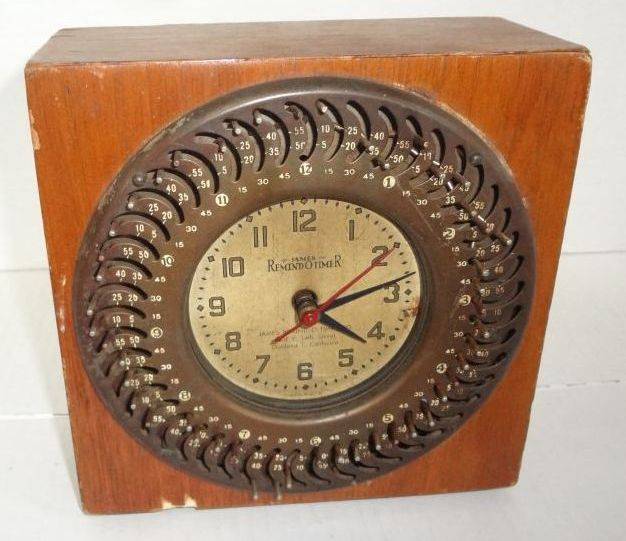This wide rectangular photograph showcases an antique remind-o-timer clock mounted on a wall consisting of white painted tiles or cinder blocks. The clock, which has seen a lot of use and displays an aged charm, is affixed to a light-to-medium brown wooden base that appears larger at the top, possibly due to the camera angle. Surrounded by a thick dark brown wooden frame adorned with intricate carved patterns, the face of the clock features a somewhat aged light brown surface. The gray numerals marking the hours (1 through 12) are prominently displayed, accompanied by smaller numbers indicative of minutes and seconds. The clock hands add further detail: the hour and minute hands are black, while the second hand is red. The clock face also prominently features the label "Remind-O-Timer," suggesting it may function as both a clock and a timer. Despite potentially being obsolete in a world dominated by smartphones, this vintage timepiece clearly serves as a decorative and nostalgic element on the stark white tiled wall.